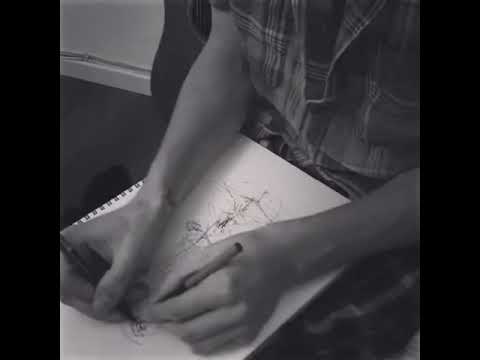In this black-and-white photo, there is a downward view of a young individual seated on the floor, drawing in a spiral-bound notepad resting on their lap. The person, whose forearms and hands are prominently featured, is using a pencil or pen in each hand, appearing to sketch simultaneously with both. Although the drawing is not clearly visible, it resembles abstract squiggles or a preliminary framework. The individual is dressed in a short-sleeved, plaid button-up shirt and pants. Surrounding details of the room suggest a bedroom setting, with visible elements such as a rug, white walls with molding, and a portion of an acoustic guitar to the side, hinting at the person's artistic inclinations. The photo's composition is bordered by thin black framing on the left and right sides, adding an interesting touch to the overall image.